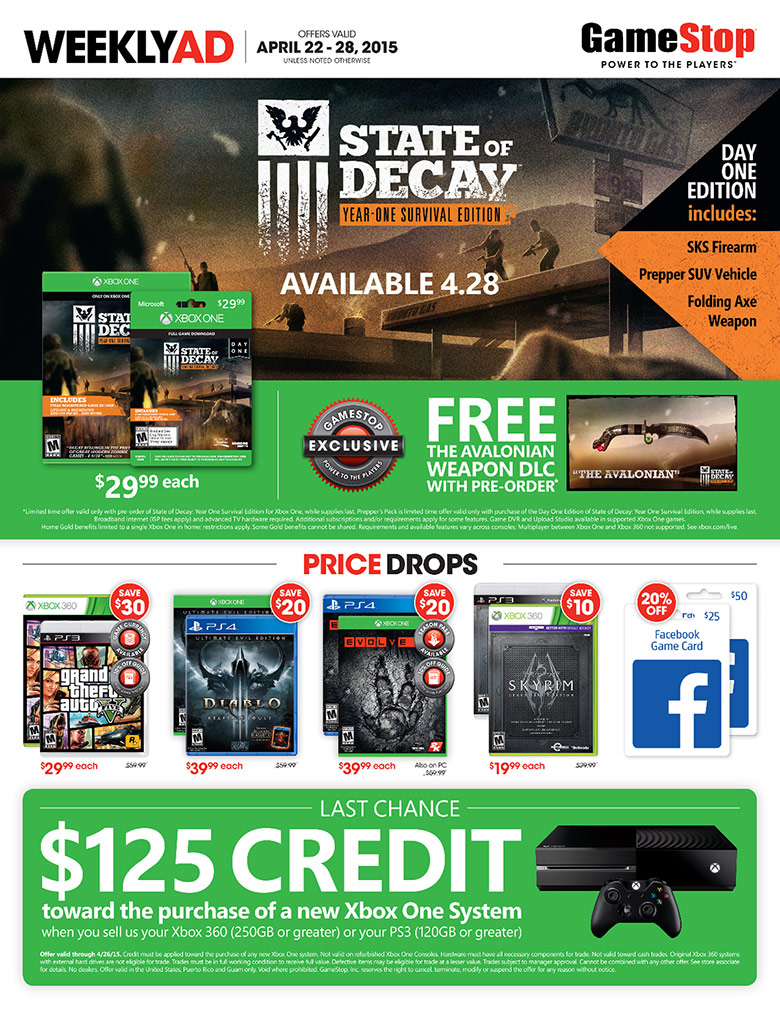The vertical rectangular image showcases a screenshot from a GameStop weekly ad, with the title at the top left reading "Weekly Ad" and the validity period "Offers valid April 22nd through 28th, 2015, unless noted otherwise." On the right side, the GameStop logo with the tagline "Power to the Players" is prominently displayed.

The top section of the ad, which is the largest and horizontally rectangular, features the "State of Decay: Year One Survival Edition." The central advertisement highlights that the game is available for $28 and includes a special offer: the Avalonian Weapon DLC for free with a pre-order, exclusively at GameStop. Additionally, the Day One Edition boasts the inclusion of the SKS Firearm, the Prepper SUV Vehicle, and the Folding Axe Weapon.

Below this main advertisement, there are five side-by-side boxes showcasing various games with corresponding discounts. From left to right:
1. "Grand Theft Auto" is advertised with a $30 savings.
2. Potentially "Diablo" offers a $20 savings.
3. The middle game is difficult to discern but mentions a $20 savings.
4. "Skyrim" is listed with a $10 discount.
5. There is a mention that Facebook game cards are 20% off.

At the bottom, there is a notable offer indicating, "Last Chance: $125 credit towards the purchase of a new Xbox One system."